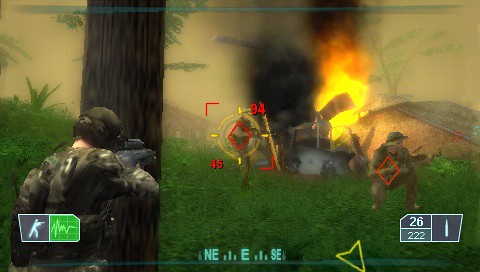In this dramatic scene from a video game, the screen captures an intense, war-torn battlefield. The sky is a smoky, golden yellow, tinged with the fires of ongoing conflict, while thick black smoke billows ominously in the background. At the forefront, an army character, clad in full military gear, stands with his back to the viewer, his posture tense and ready. He aims his gun precisely, fixating on a diamond-shaped target marker hovering over another distant player. The bottom of the screen displays essential interface elements: a compass for navigation, indicators for various possible movement directions, and crucial information regarding the player's health status. The visual chaos and the meticulously detailed interface combine to immerse the viewer in this high-stakes, action-packed moment of digital warfare.